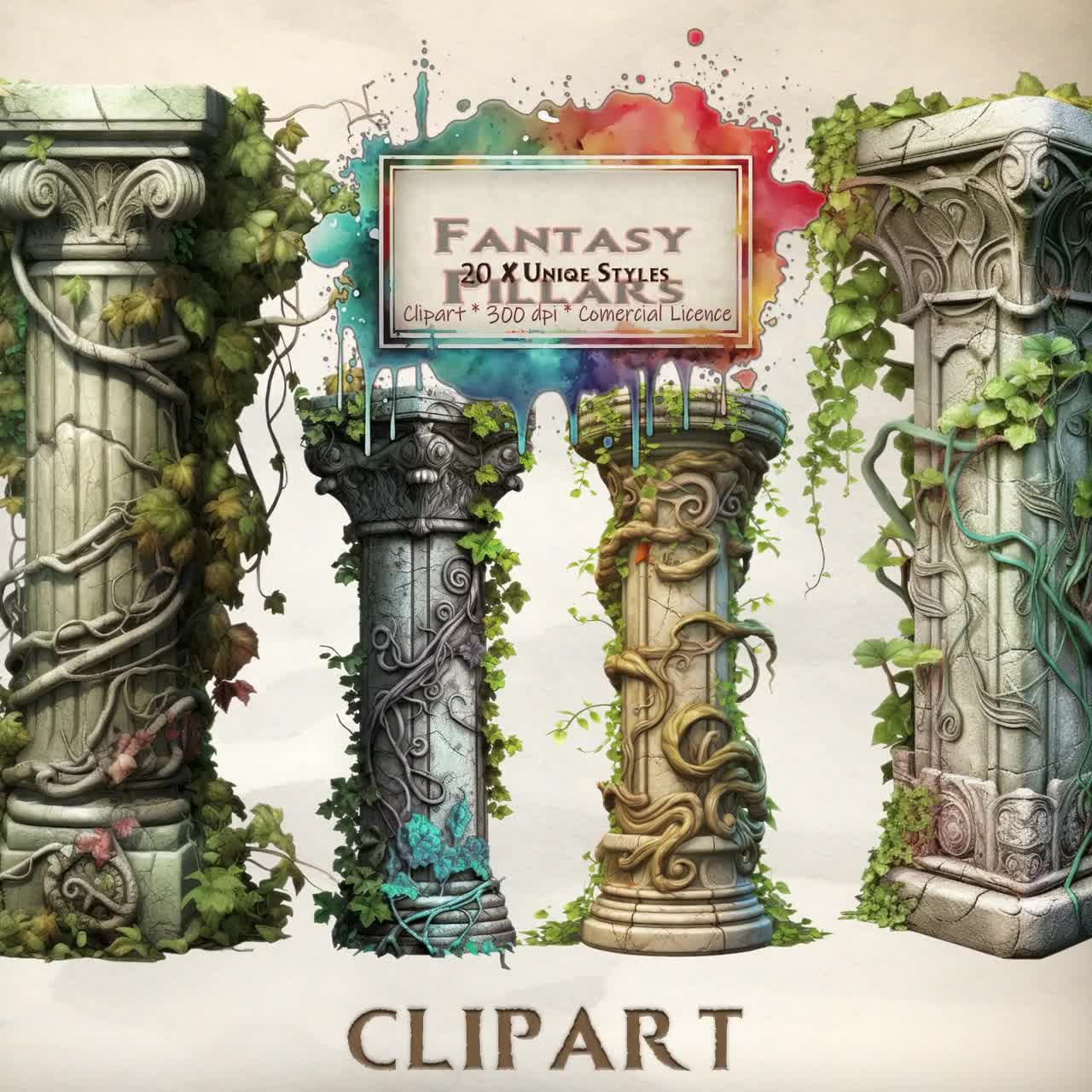This computer-generated clip art image features an off-white background with four intricately detailed columns adorned with green ivy and vines. The two large columns on the sides have expansive vine growth, while the two shorter columns in the middle show similar embellishments, with one column appearing gray and the other white. The leftmost column is specifically noted to be white, and blue flowers are entwined around the bottom of the shorter middle column. Above the columns, there is text, seemingly spray-painted, that reads "Fantasy Pillars," along with "20x Unique Styles, Clip Art, 300 DPI, Commercial License"—note that ‘Commercial’ is misspelled with a single ‘m’. Below the columns, additional text in brownish-gray capital letters on a white background states "Clipart." This elaborate artwork combines multiple elements and includes detailed labeling for commercial use.